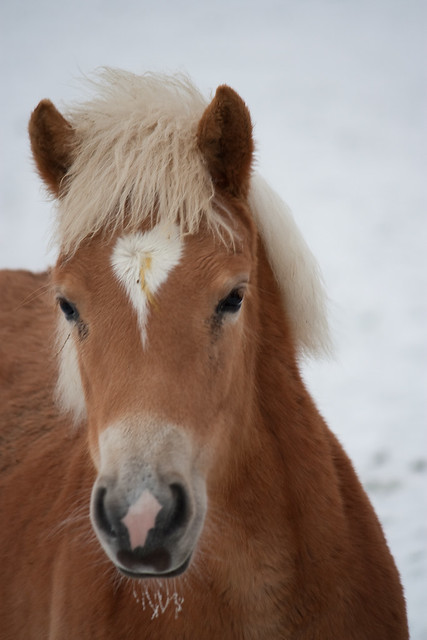In the foreground of a snowy winter scene, a Shetland pony stands with its head slightly left of the center. The pony's dense fur is an auburn or brownish-red color, contrasting vividly against the white snow. Its mane is a distinctive blondish-cream and has a comical mullet-like appearance, with shorter bangs and longer sections on the sides. Poking through the mane are two brown ears that match the fur of its body.

The pony's expressive black eyes look out from beneath this mane. A heart-shaped white patch adorns its forehead, adding a charming detail to its visage. The snout is multicolored, starting with white fur above, a noticeable pink spot in the middle, and ending in black around the nostrils and lips. The pony's whiskers below its mouth are tipped with tiny icicles, evidence of the cold climate.

The background emphasizes the wintery setting, with a grayish sky above and the ground covered in a blanket of white snow. Some black rocks can be seen, blurred in the distance, adding depth to the image. Overall, the scene vividly showcases the pony braving the cold, its detailed features standing out against the stark, snowy backdrop.